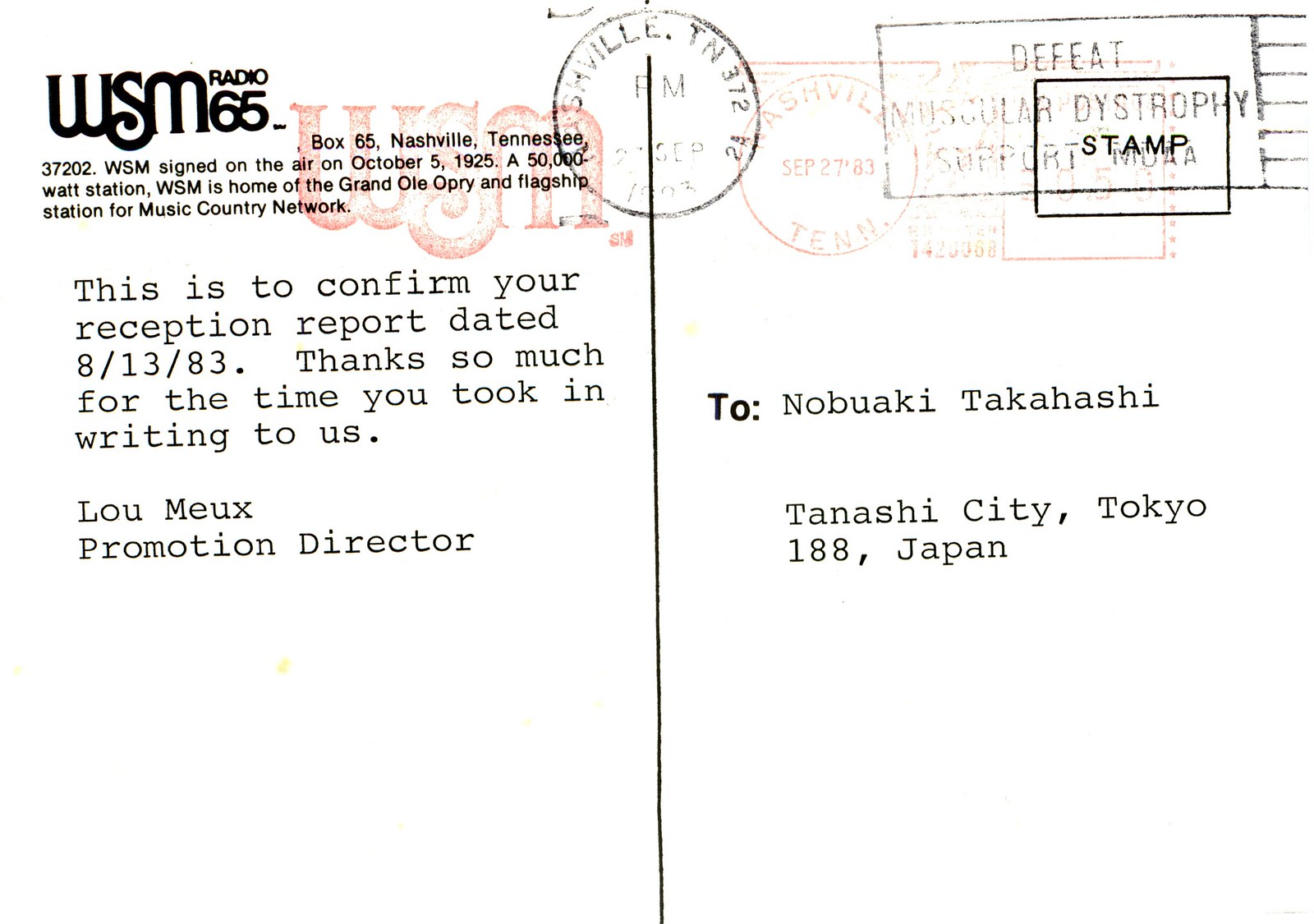The back of a postcard is slightly tilted to the left and prominently features various stamps and text. In the upper left corner, in dark black letters, it says "WSM Radio 65," with a red stamp overlapping the text, also marked "WSM." To the right of this, there is a faded mail stamp reading "Nashville, Tennessee 327 24 PM." Additional post office stamps from different stops are scattered nearby. On the right side of the postcard, there is an address: "To: Nobukawa Takahashi, Tanashi City, Tokyo, 188, Kama, Japan." On the left side, below the "WSM Radio 65" header, an elaborate inscription details: "Box 65, Nashville, Tennessee 37202. WSM signed on the air October 5th, 1925, as a 50,000-watt station. WSM is home of the Grand Ole Opry and Flagship station for the Music Country Network." Underneath this historical note, another typewritten message reads: "This is to confirm your reception report dated 8/13/83. Thanks so much for the time you took in writing to us. Lou Moe, Promotion Director." A thick black line in the center splits the left side’s descriptive notes from the right side’s address details.